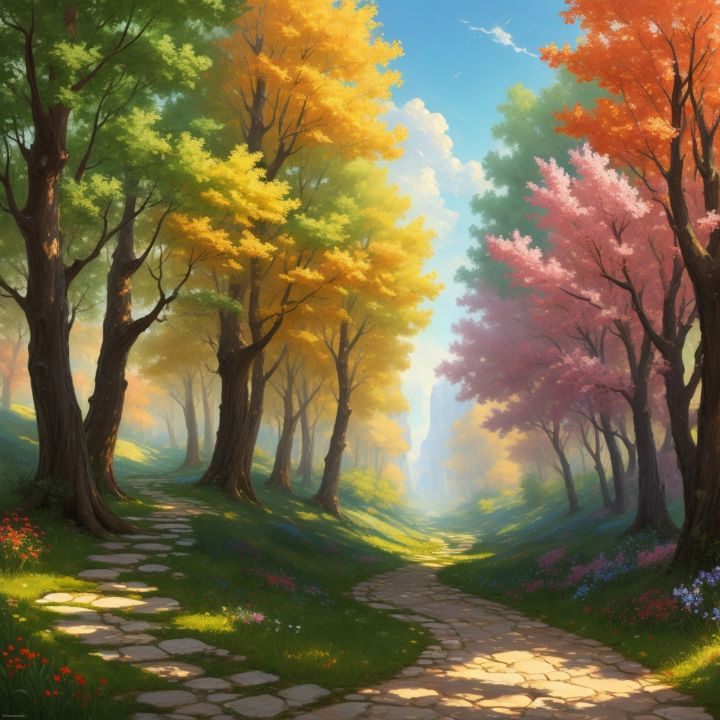A vibrant digital image captures a picturesque scene of two winding stone pathways cutting through a lush, garden-like forest setting in the fall. The primary pathway, composed of light beige stones, curves to the right, then left, and back to the right, flanked by lush green grass on either side. Parallel to it, another path veers to the left, also edged with lush greenery and wildflowers in shades of white, yellow, red, pink, and blue.

Towering trees create a canopy of varied hues, displaying leaves that transition from greens and yellows on the left side to oranges, pinks, and some lime greens on the right. The interplay of colors resembles an almost gradient effect, suggesting a seasonal transformation. The bright yellow, orange, and pink leaves contrast vividly against the verdant landscape. The scene is illuminated by a sunny day with scattered clouds, casting a warm light over the serene environment. This tranquil setting, devoid of people or animals, exudes a serene, almost dream-like quality that blends natural beauty with artistic charm.